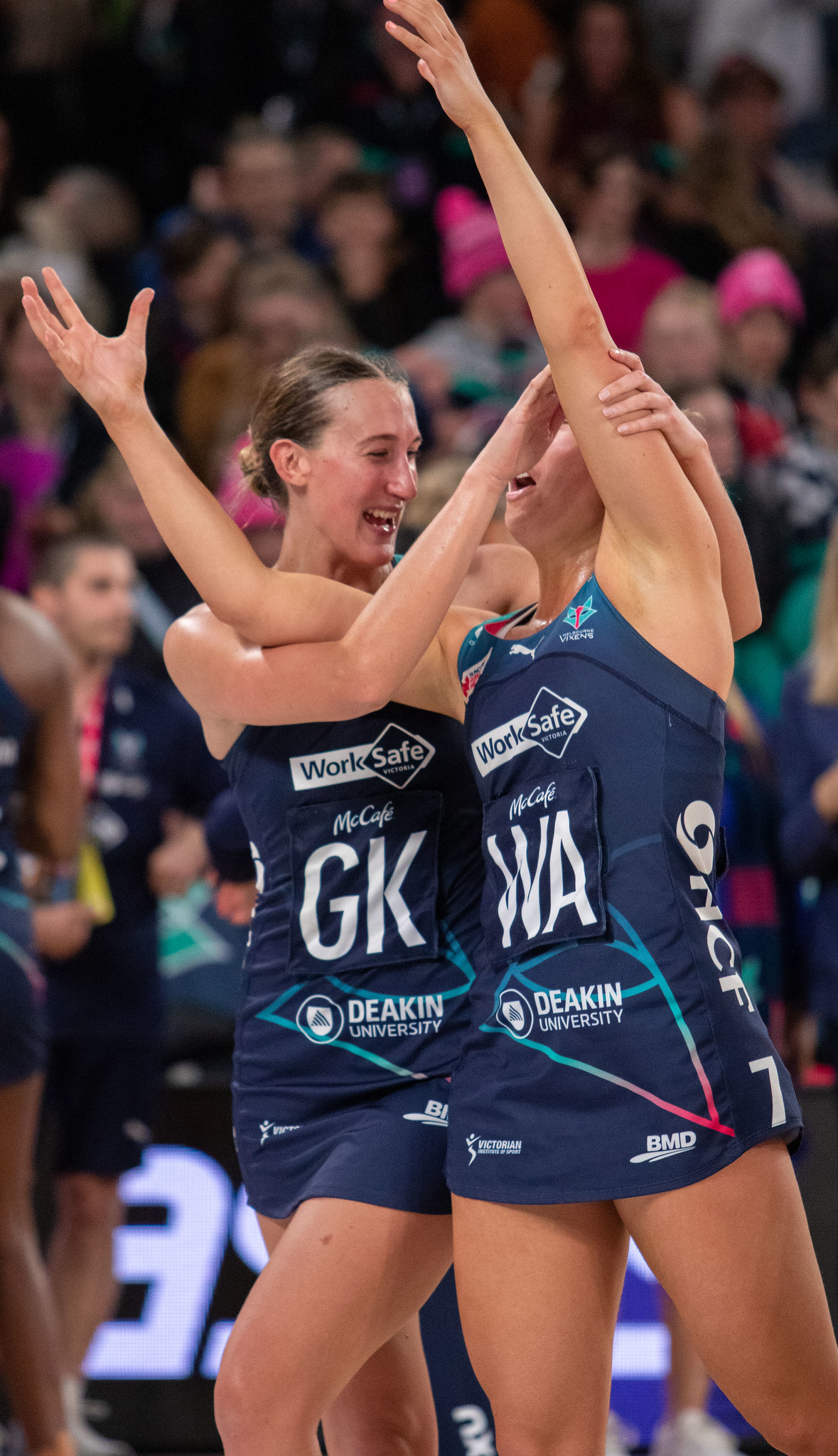In this vibrant photograph taken at an athletic championship, two women are prominently featured, appearing to celebrate a recent triumph. Both women, dressed in navy blue sleeveless tunics that resemble athletic uniforms, showcase several sponsorship emblems, including "Work Safe," "McCafe," and "BMD," along with "Deakin University" logos. The woman on the left has her arms triumphantly raised in the air, her hands open, while the woman on the right, identified by the large initial "WA" on her uniform, is smiling broadly and has her arm draped affectionately across her partner, whose uniform bears the initials "GK." The sporting venue in the background is filled with an out-of-focus crowd, many wearing pink hats or beanies, adding to the festive, celebratory atmosphere. The scene exudes joy and achievement, capturing a moment of shared excitement and camaraderie within the competitive setting.